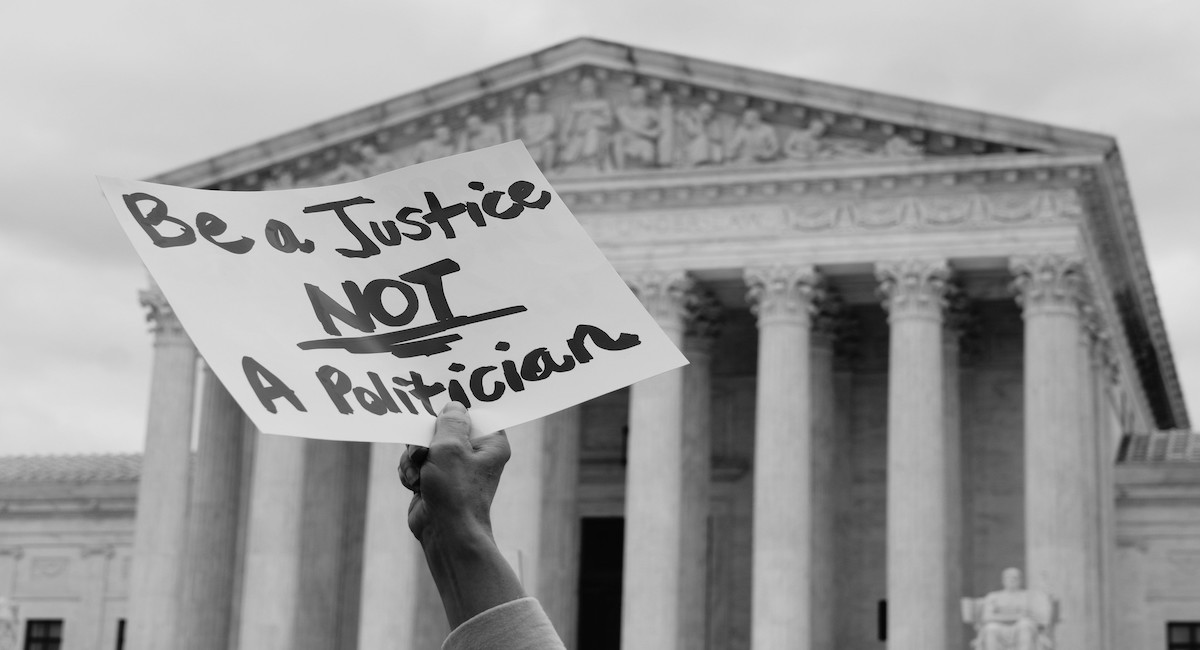This black-and-white photograph captures a protest scene in front of what appears to be the United States Supreme Court building. Dominating the foreground is a dark-complected hand emerging from the bottom of the image, holding a white sign with a powerful message written boldly in black Sharpie. The sign reads, "Be a Justice, Not a Politician," with the word "NOT" emphasized in all caps and heavily underlined. The hand, clad in a white sleeve, is the only visible sign of human presence in the image. In the background stands the imposing Greek Revival architecture of the Supreme Court, characterized by its grand neoclassical facade, rows of tall Roman-style columns, and a pitched roof adorned with intricate stone carvings, including statues. The sky above is dotted with clouds, casting a dramatic backdrop to the protest.